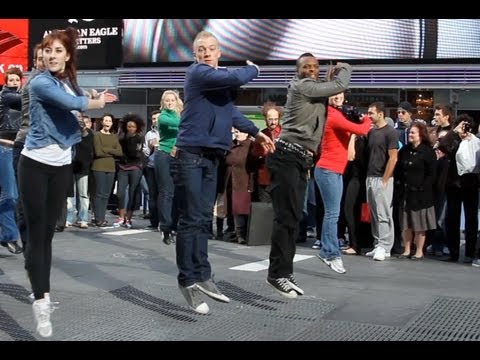This vibrant color photograph captures a close-up shot of a flash mob performing a meticulously synchronized dance routine in a shopping mall. The scene is set in front of a large billboard advertising American Eagle Outfitters. Six dancers form the core ensemble, with four prominently featured in the front row: a white woman on the far left rising on her left toe, a white man next to her who is slightly off the ground mid-jump and looking directly at the camera, a black man who is also airborne, and another white woman whose face is partially obscured by the second man's right arm but shows a hint of a smile. All participants are dressed casually in t-shirts, jeans, and sneakers, adding a spontaneous feel to the performance. Behind them, two more white women enhance the symmetrical choreography. The dancers are captured in mid-motion, each extending their right arms in near-perfect unison as they look to their right, creating an illusion of effortless coordination. Encircling the dancers, a crowd of onlookers beams with amusement and enjoyment, all eyes fixated on the dynamic scene unfolding before them.